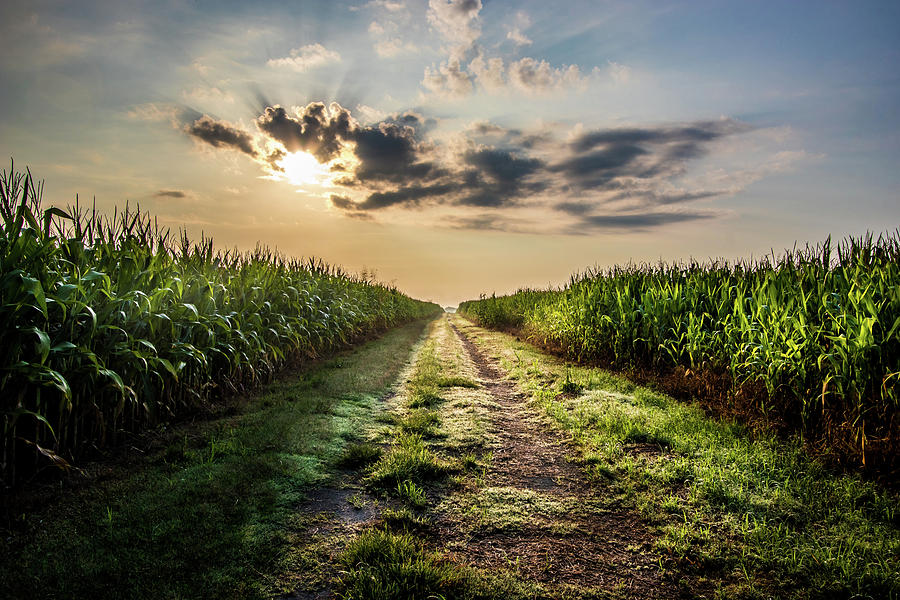The photograph depicts a serene farm road that stretches from the foreground to a vanishing point near the middle of the image, flanked by tall rows of corn on both sides. The road, primarily intended for off-road vehicles and tractors, features a grassy middle flanked by two dirt tracks, indicating minimal vehicular traffic. The corn, dark green and adorned with tassels, appears to be thriving, suggesting it is either late spring or summer. The sky above is a dramatic mix of blue, white, and gray clouds with a significant dark cloud sitting prominently in the middle. The sun, positioned towards the upper left, is partially obscured by the clouds, emitting a soft, diffused light that casts a light green hue on some of the corn while leaving the rest in shadow. The horizon is tinged with hues of yellow-orange and light pink, contributing to the impression that the photograph was taken at dusk, as the sun sets, shrouding the scene in a gentle, picturesque light.